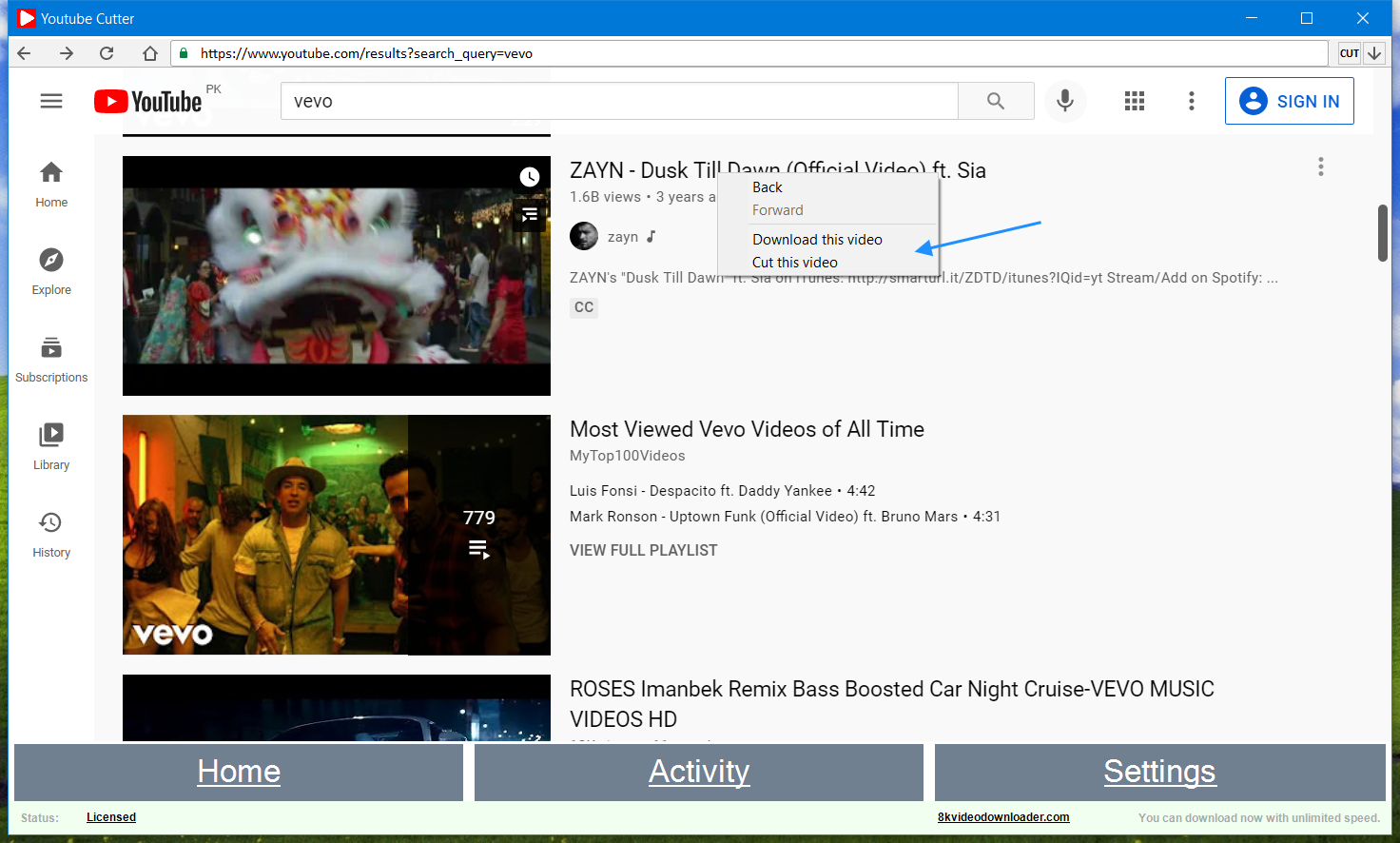A screenshot of a specialized browser interface within the "YouTube Cutter" application is displayed. At the top, there's the URL bar which reads "youtube.com" and features a down arrow next to the text "out." Positioned below the URL bar is the YouTube website indicated by a recognizable red circle logo.

The screen prominently features a YouTube page displaying the "Zayn - Dusk Till Dawn (Official Video) ft. Sia" with a blue arrow pointing towards the option to "cut this video" upon right-clicking. Additional sections on the page include "Most Viewed Vevo Videos of All Time" and "Roses in Moundback Remix (Bass Boosted) - Karanay Cruz," showcasing various video options.

At the bottom of the screen, there’s a gray horizontal navigation bar with options labeled "Home," "Activity," and "Settings" in white text. A notice also appears indicating users can "download now with unlimited speed." This detailed interface implies the app allows users to browse YouTube and cut or edit segments of videos directly within the app's environment, although the exact functionalities remain unclear.